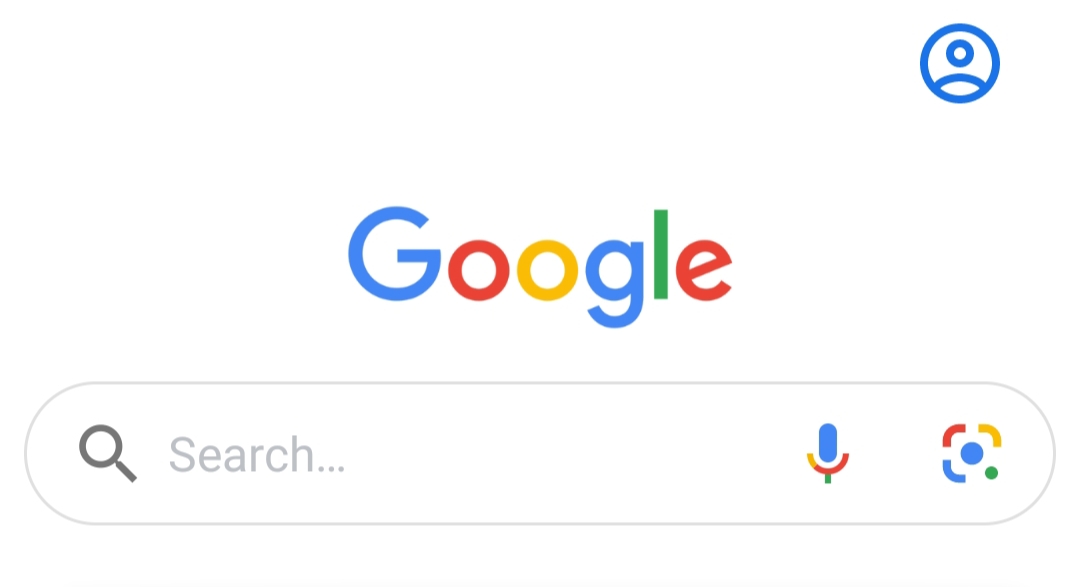The image depicts the top section of the Google search page set against a white background. Located at the upper right-hand corner is a distinctive circular profile icon, characterized by a blue outline and a white interior. Within this circle, there is a small, centered silhouette representing the user's profile. Below this is the iconic Google logo prominently displayed in the center of the page. The logo features a capital "G" in blue, followed by a lowercase "o" in red, another lowercase "o" in yellow, a lowercase "g" in blue, a lowercase "l" in green, and a lowercase "e" in red. Directly underneath the Google logo lies the familiar Google search bar, waiting for user input.